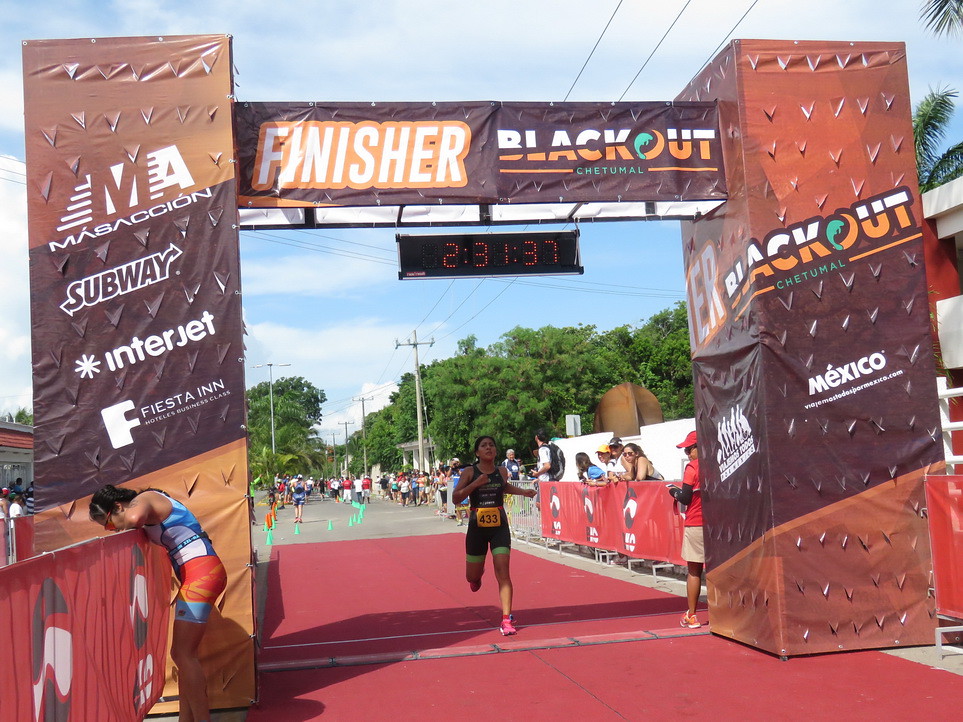The photograph captures a bright, sunny day at the finish line of a race, likely a marathon, with a vivid blue sky dotted with fluffy white clouds. Central to the scene is a tall, arch-like structure that frames the finish line, adorned with sponsor logos including Blackout, Fiesta Inn, Interjet, Subway, and likely others, alongside a prominent "Finisher" banner. A digital clock above the arch shows the time "2:31:37" as runners complete the race. To the left, a female runner, seemingly exhausted, is bent over a half-fence, perhaps catching her breath or feeling unwell. At the center, a male runner, donned in black running gear with the number 433 on his jersey and pink shoes, is about to cross the red-carpeted finish line. Nearby, a photographer stands to the right, capturing the moment. Spectators line both sides of the finish area, cordoned off with bright green pylons, and trees flank the road that continues beyond the finish line, populated with more runners and onlookers.